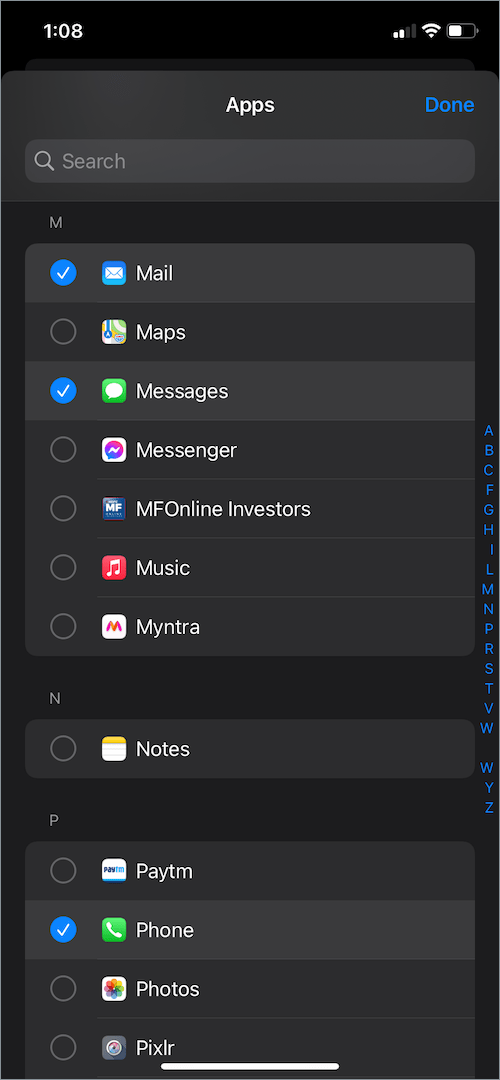Portrait-format screenshot displaying a smartphone interface in color. The time displayed is 1:08 (either AM or PM, non-military time). The battery is at approximately 50%, with the device showing full internet connectivity with three bars and two out of four bars for 3G data. The screen shows the app selection menu where several applications are listed: Mail (likely Outlook), Maps, Messages, Messenger, MFonline Investors, Music, Mintra, Notes, Paytm, Phone, Photos, and Pixlr. Notably, Mail, Messages, and Phone are highlighted with tick marks, indicating they are selected.